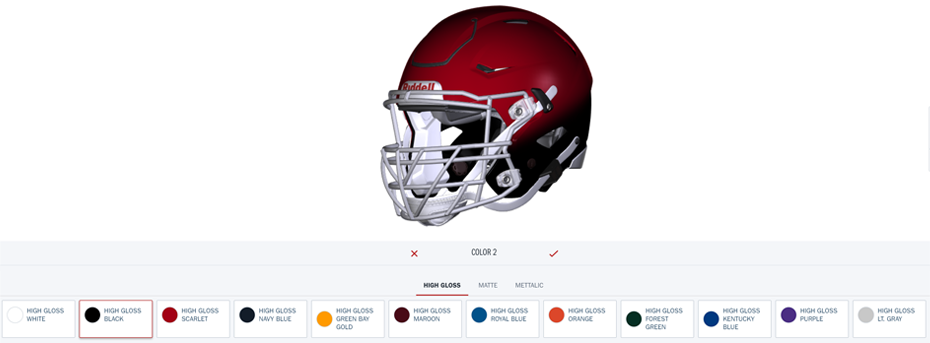The image depicts a football helmet customization page from an online store, prominently displaying a maroon Riddell helmet. The helmet is available in a variety of high gloss colors including white, black, scarlet, navy blue, baby blue, green, maroon, royal blue, orange, purple, forest green, light gray, and Kentucky blue. Above the helmet, a dropdown menu allows users to select among different colors, with black currently selected and visible on the helmet's lower part. Additional navigation options include unselected "Matte" and "Metallic" finishes, with "High Gloss" being the chosen finish. Other interface elements include an X and a check mark for navigating through sections or closing the page.